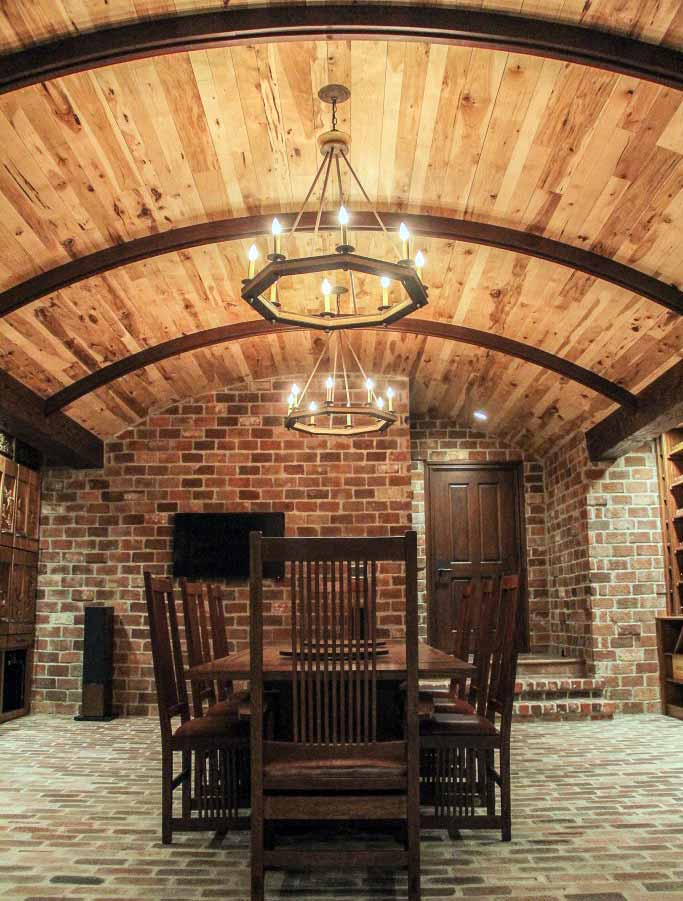This realistic, horizontally oriented photograph depicts an atmospheric cellar or cabin. The room is characterized by its red and brown brick walls and floor, creating a warm, rustic ambiance. Its arched wooden ceiling, reminiscent of a barrel's interior, is supported by arched metal beams and wooden planks. Dominating the center of the space is a large, rectangular dark wood table surrounded by eight matching wooden chairs, all bathed in the soft glow of two simple chandeliers with candle-like lights. On the far right, there's a substantial oak door, adjacent to built-in wooden shelving. The ceiling features long, dark wooden beams stretching across its length. The image is well-lit from the chandeliers and contains no text, emphasizing its visually rich, traditional style.